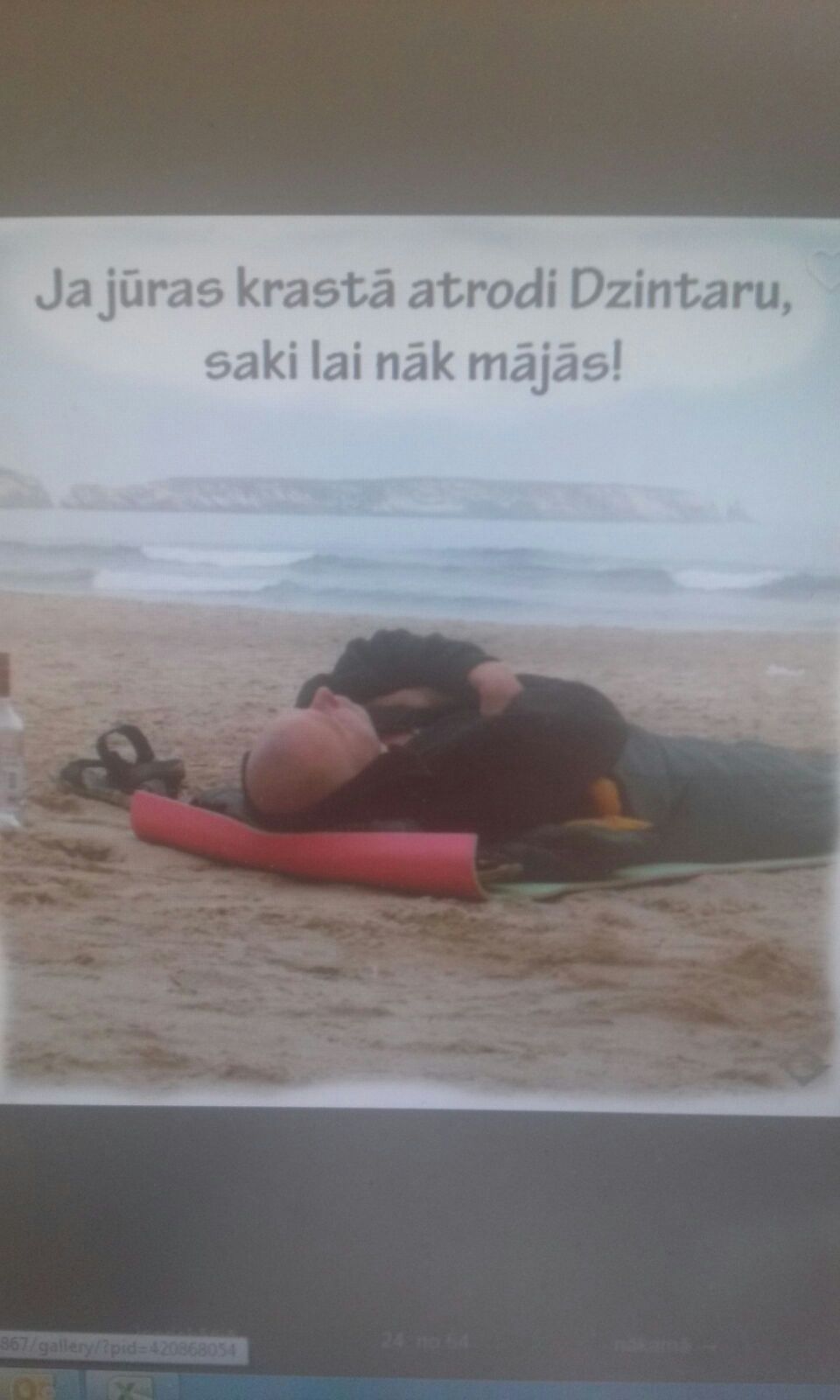The image captures a photorealistic scene of a bald man resting on the golden sand of a beach. He is lying on a mat that has a green top and red bottom, positioned with his head towards the left and his feet to the right. The man is wearing a blue or black jacket and gray pants, with his arms crossed over his chest, giving the impression that he might be sleeping. Near him, on the left side, there's a clear bottle and a single brown sandal. In the background, blue waves can be seen rolling onto the shore, and a large dark blue landmass is visible on the horizon line. Above the ocean, a blue sky with a large white cloud-like shape is present, over which text in another language is written in dark gray. The entire scene is observed through a computer screen, evident by the visible blue taskbar at the bottom displaying different apps like Excel.